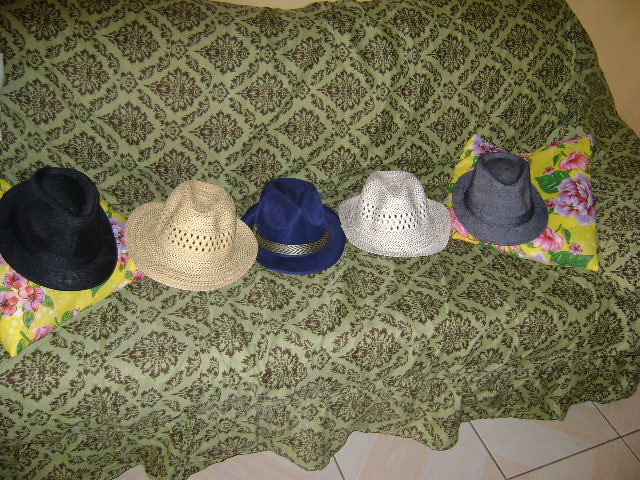The image depicts an old-fashioned, regular-length sofa draped with a light green throw cover adorned with a reddish-brown diamond and scroll design, giving it a vintage appearance. The sofa features two yellow floral throw pillows with vibrant pink and purple flowers and green leaves—one on each end of the sofa. Lined up neatly across the sofa are five hats. On the leftmost throw pillow rests a black hat with a matching black brim. Next to it is a beige straw hat with a wide brim and perforated details around the crown. The third hat is navy blue with a black and silver band around it. The fourth hat, made of white straw, mirrors the beige hat's style but is white in color. Finally, on the right throw pillow sits a gray hat that resembles the black one on the other end, complete with a matching gray brim and ribbon. The sofa is situated over a large beige tile floor, and the hats are displayed as if for a showcase.